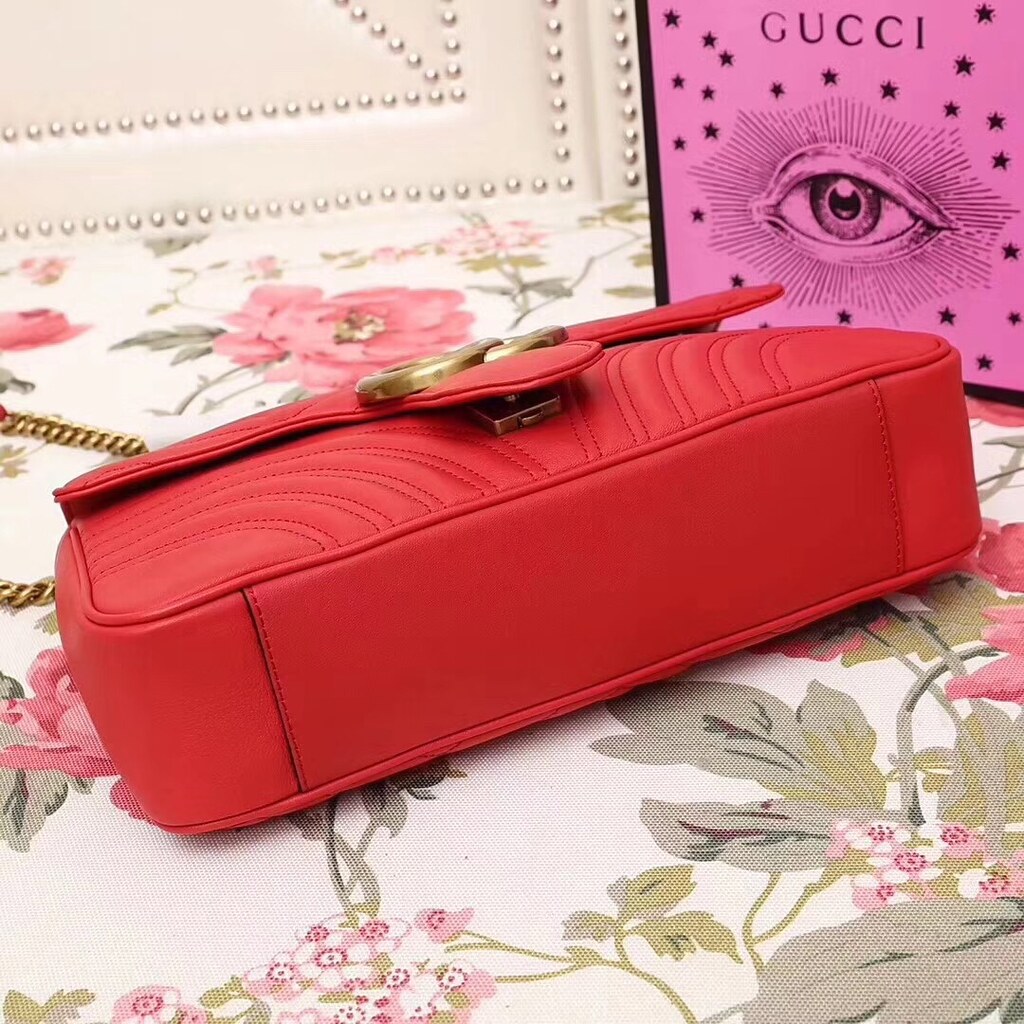This professional square color photograph showcases a luxurious, red leather Gucci handbag positioned diagonally in the center of the image. The handbag, which is slightly smaller than average, is visually striking with its bold red hue and intricate stitching. A shiny gold badge, likely featuring the Gucci logo, adorns the front and is attached to a brass-colored chain shoulder strap. The handbag is placed on a patterned cloth featuring pink flowers with green leaves and stems, as well as additional floral details in white and gray. In the upper left corner, part of another studded fabric item is visible. To the top right, there's a prominently placed pink Gucci placard, featuring an eye surrounded by rays and black stars, with the Gucci logo at the top, enhancing the luxurious and artistic presentation of the scene. This image boasts professional clarity, focus, and lighting, emphasizing the refined details of the handbag and its elegant surroundings.